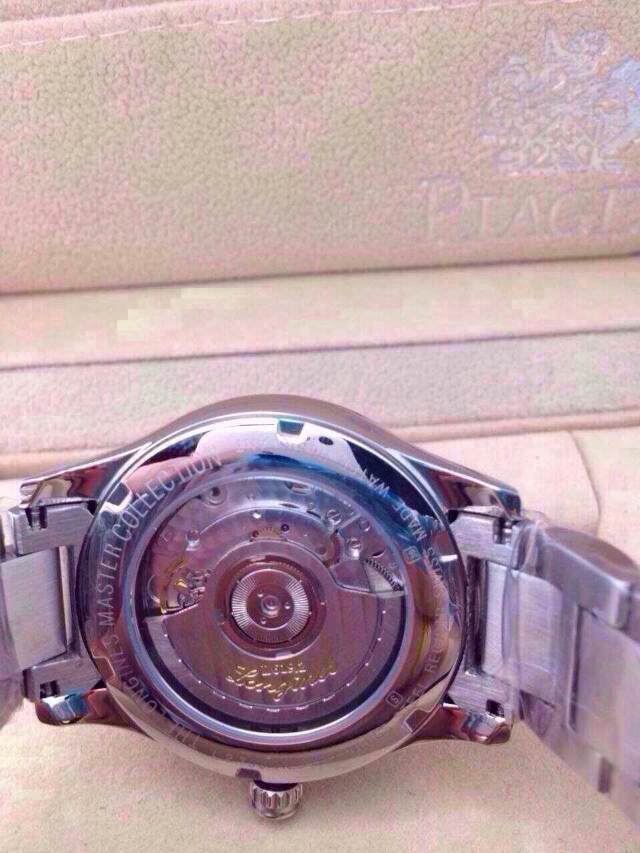This color photo captures the detailed back of a silver men's wristwatch, exhibiting a steel gray metal band composed of interlinked clasps. The clear, see-through back case reveals an intricate view of the watch's inner gears, hinting at a traditional wind-up mechanism. Gold and white inscriptions are present, with partial text decipherable as "Master Collection" and possibly "Made in the States." Additionally, a signed date is subtly etched on the back. The watch rests on a surface that appears to be either a tan leather material or a peach-colored sofa. Accompanying the watch, a distinctive box featuring a mixed pink and beige camouflage pattern is visible, marked with a logo starting with "P-I-A-C-E" at the top.